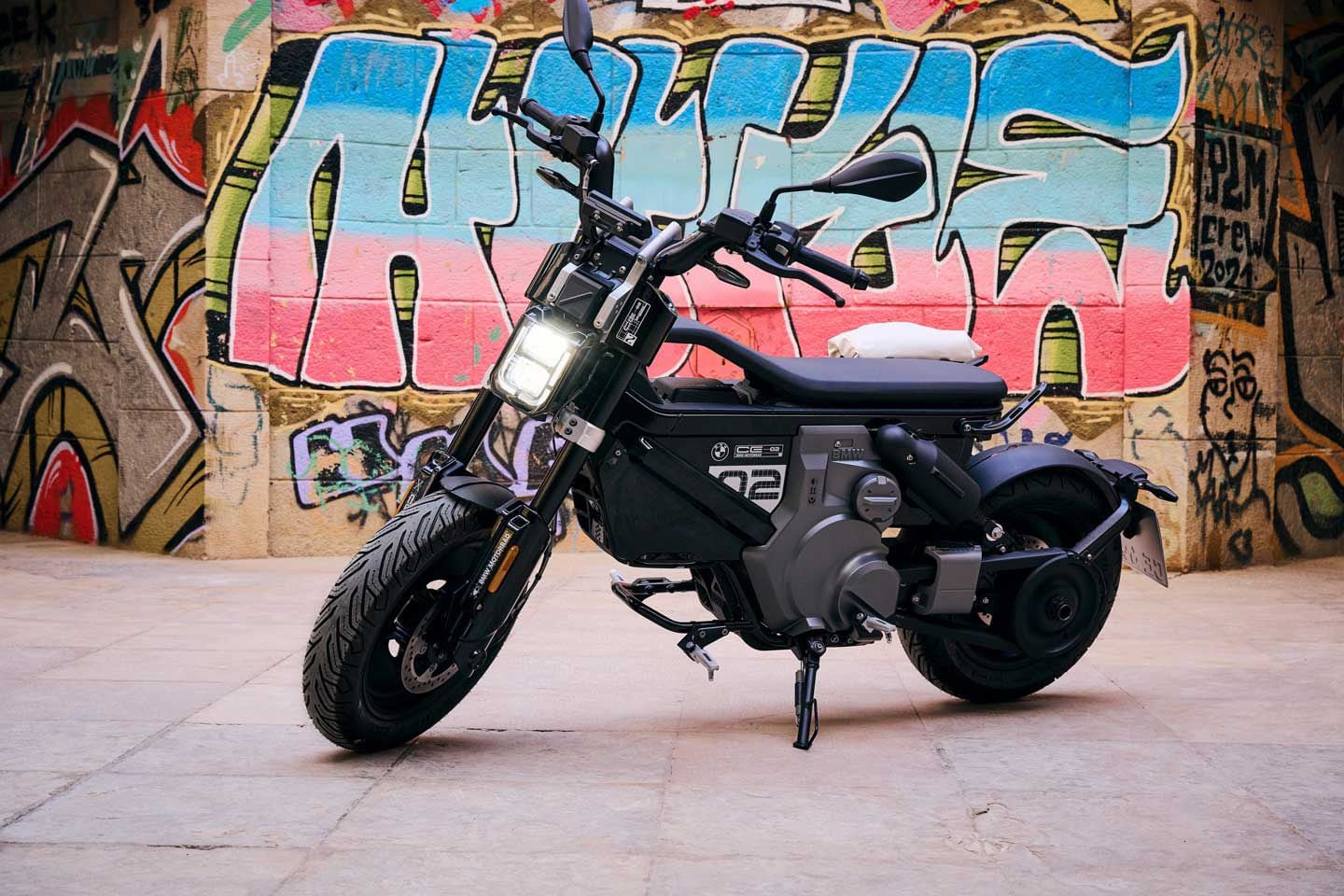This photograph features a black BMW motorcycle with silver accents, parked with its kickstand down and its headlight on. The bike displays a bold "02" stenciled on its side, suggesting a potential racing association or model identification. The motorcycle, which has a futuristic design, is equipped with what appears to be an electric battery instead of a traditional gas tank, as inferred from the absence of a gas tank. A BMW logo is visible on the motorcycle, further confirming its make.

The backdrop of the image is a heavily graffitied wall located in an outdoor setting. Prominent in the graffiti is a colorful piece that transitions in a gradient pattern from robin's egg blue at the top to deep pink and red at the bottom. One piece of graffiti boldly declares "Crew 2021" in black ink. The wall is adorned with a variety of bubble letters and sketches, contributing to a vibrant and chaotic urban aesthetic. The numerous shades of blue, light pink, and dark pink, along with other assorted colors, add a dynamic splash to the overall scene. A license plate can also be seen hanging from the motorcycle's back fender.